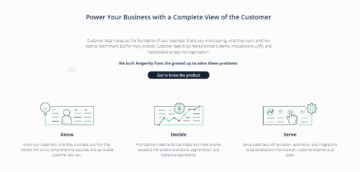In this small, blurry image, we can discern several elements despite the lack of clarity. At the top middle, there is a bolded text in black reading, "Power your business with a complete view of the customer." Directly below this, a passage of text appears, resembling a paragraph, although it is illegible due to its smaller font size compared to the bold heading above. Further down, another set of bolded words states, "We built the read up the problems." Proceeding this text, there is a distinct black rectangle with white text inside that likely says, "Get to know the product."

The bottom half of the image is divided into three categories. On the bottom left, within a rectangular frame, there is an image of a person's body flanked by horizontal bars on both sides. The center category, also rectangular, showcases these horizontal bars as well, but includes an additional graph-like image. The final section on the bottom right features a hand pressing a button, with the familiar horizontal bars present in the background.